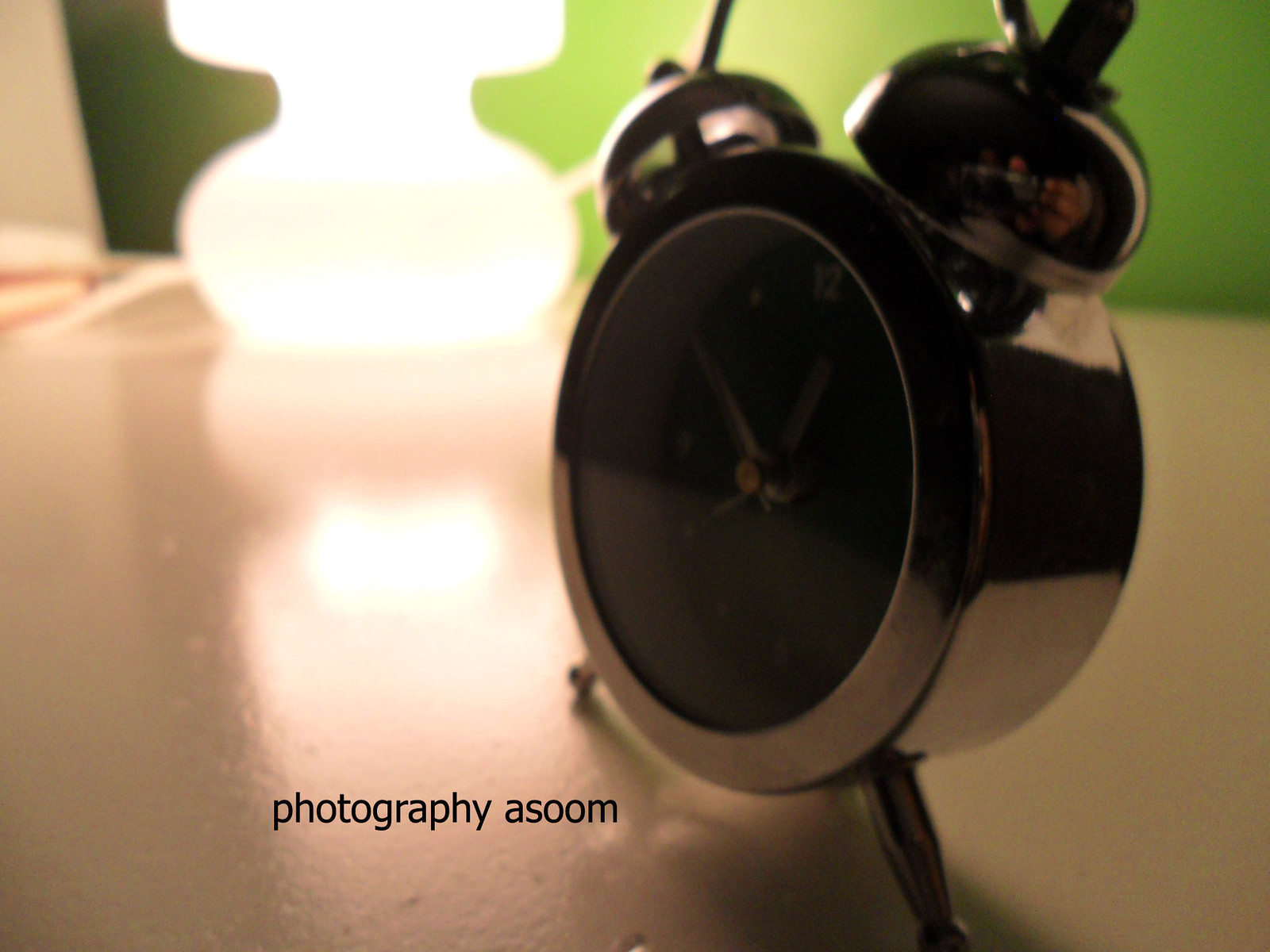The photo features a close-up of an old-fashioned, dark bronze travel alarm clock with two bells on top. The clock's face is black and distinguished by faint, metallic hour and minute hands that match the clock's bronze body, and a second hand pointing to the number 7. The clock reads 12:50. Propped up on two small brass legs, the clock rests on a cream-colored surface, possibly a table. In the background, a silhouetted, hourglass-shaped white lamp is visible against a lime green wall, adding depth to the composition. At the bottom left corner, the text "Photography ASOOM" is prominently displayed.